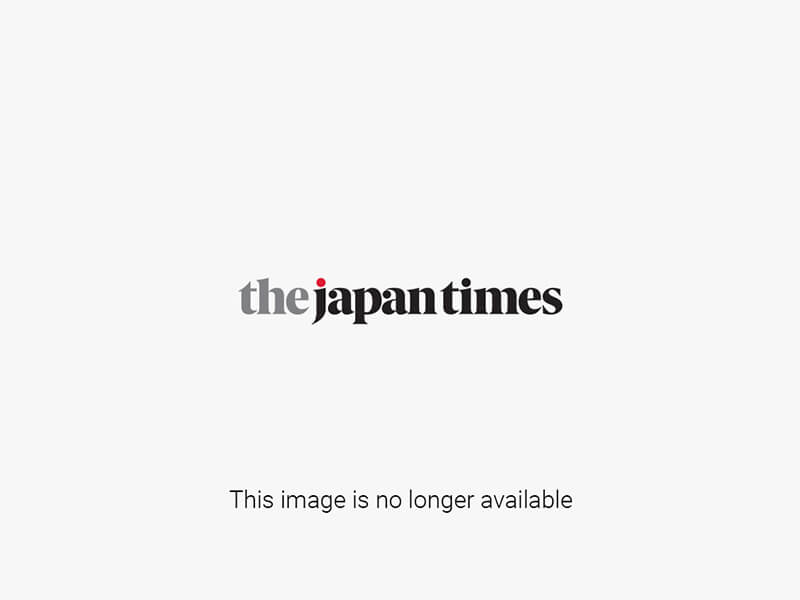The photograph captures a dynamic scene of a girl deeply immersed in karate practice. She has light, clear skin and dark eyes. Her dark hair is pulled back, revealing a determined expression with her mouth slightly parted, as she looks up and to her left, possibly at an opponent or instructor. Dressed in the classic white karate gi with a black belt, her right fist is held close to her chest while her left arm extends outward in a striking pose. This stance illustrates her proficiency and dedication to karate, emphasizing her role as both a practitioner and a potential instructor. Standing between two men, she commands attention; the man to her left gazes at her intently, his stature matching hers, while the taller man to her right stands at attention, hands crossed, and displaying a belt with a "K" inscription. The scene is set against a backdrop featuring a blue and orange metal gate, with a string tied and extending to the top of the picture, adding to the ambient training environment.